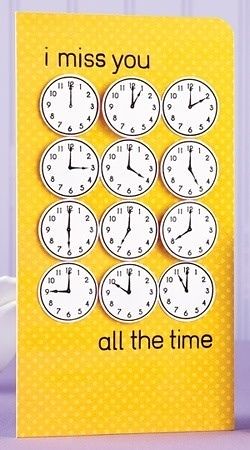This detailed description can be formulated into the following caption:

"Greeting card featuring an intricate design on a lilac or light purple textured background, resembling crumpled fabric. Central to the design is a vertically oriented yellow rectangle adorned with a subtle pattern of lighter yellow, hexagonally close-packed dots. Positioned on this rectangle are 12 clocks, arranged in four rows of three, each displaying a different hour from the 12-hour clock cycle, starting at 12 and advancing through to 11. Above the clocks, a heartfelt message reads 'I miss you,' while below them, the sentiment is completed with 'all the time.' The clocks, with their white faces and black hands, add a timeless touch to this elegant card."